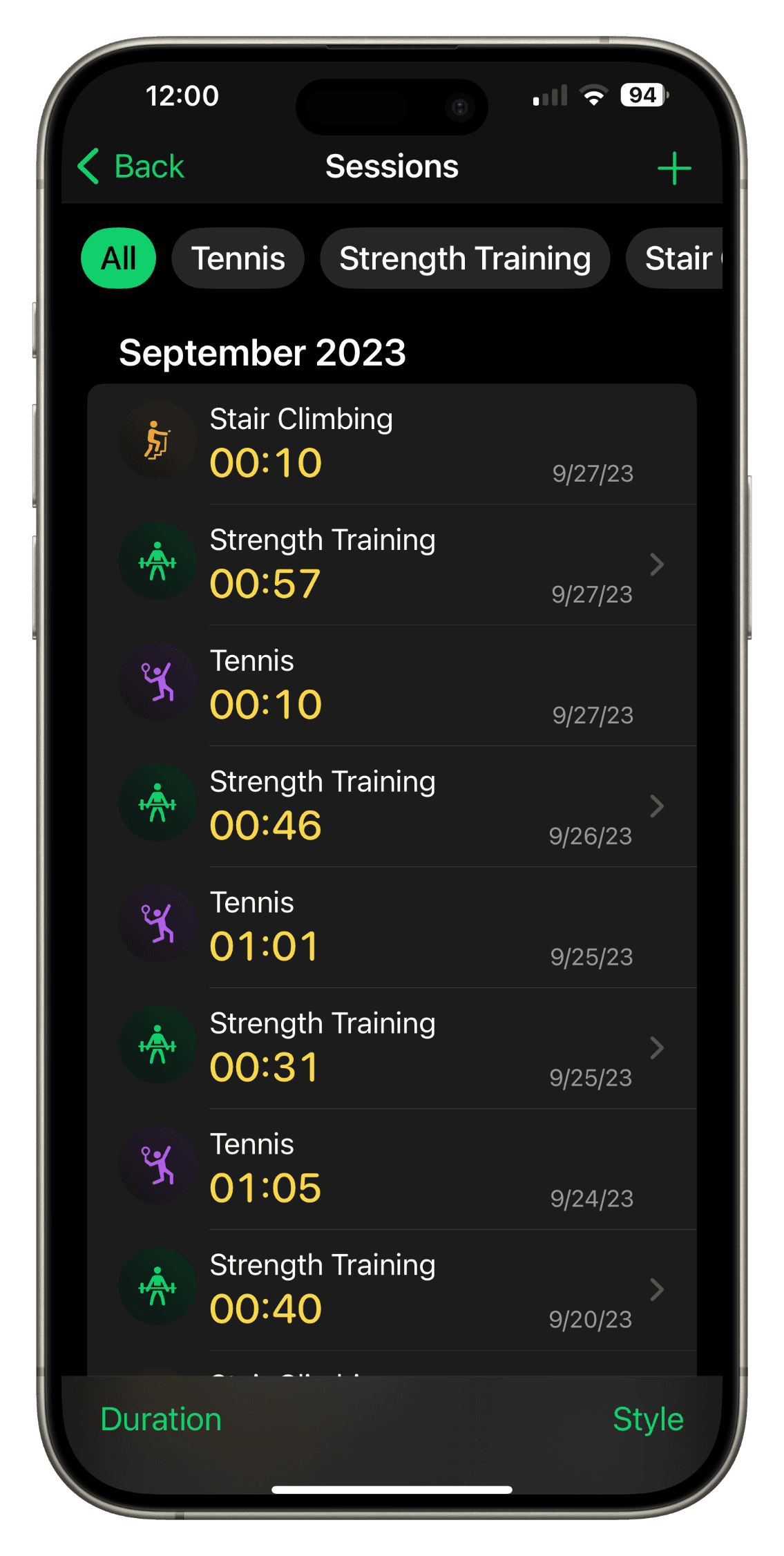A screenshot of a fitness app displays various workout sessions. At the top left, the screenshot captures the time as 12:00, while the top right corner shows icons for data, Wi-Fi, and a battery level at 94%. In the center of the screen, the heading "Sessions" is visible. The app features different workout categories, including tabs for Tennis, Strength Training, and Stair Climbing, though some tabs are cut off. The main display lists sessions for September 2023 with detailed durations: Stair Climbing for 10 minutes, Strength Training for 57 minutes, Tennis for 10 minutes, more Strength Training for 46 minutes, Tennis for 1 hour and 1 minute, another Strength Training for 31 minutes, Tennis for 1 hour and 5 minutes, and another Strength Training session for 40 minutes. The word "Style" is seen at the bottom right of the screenshot.